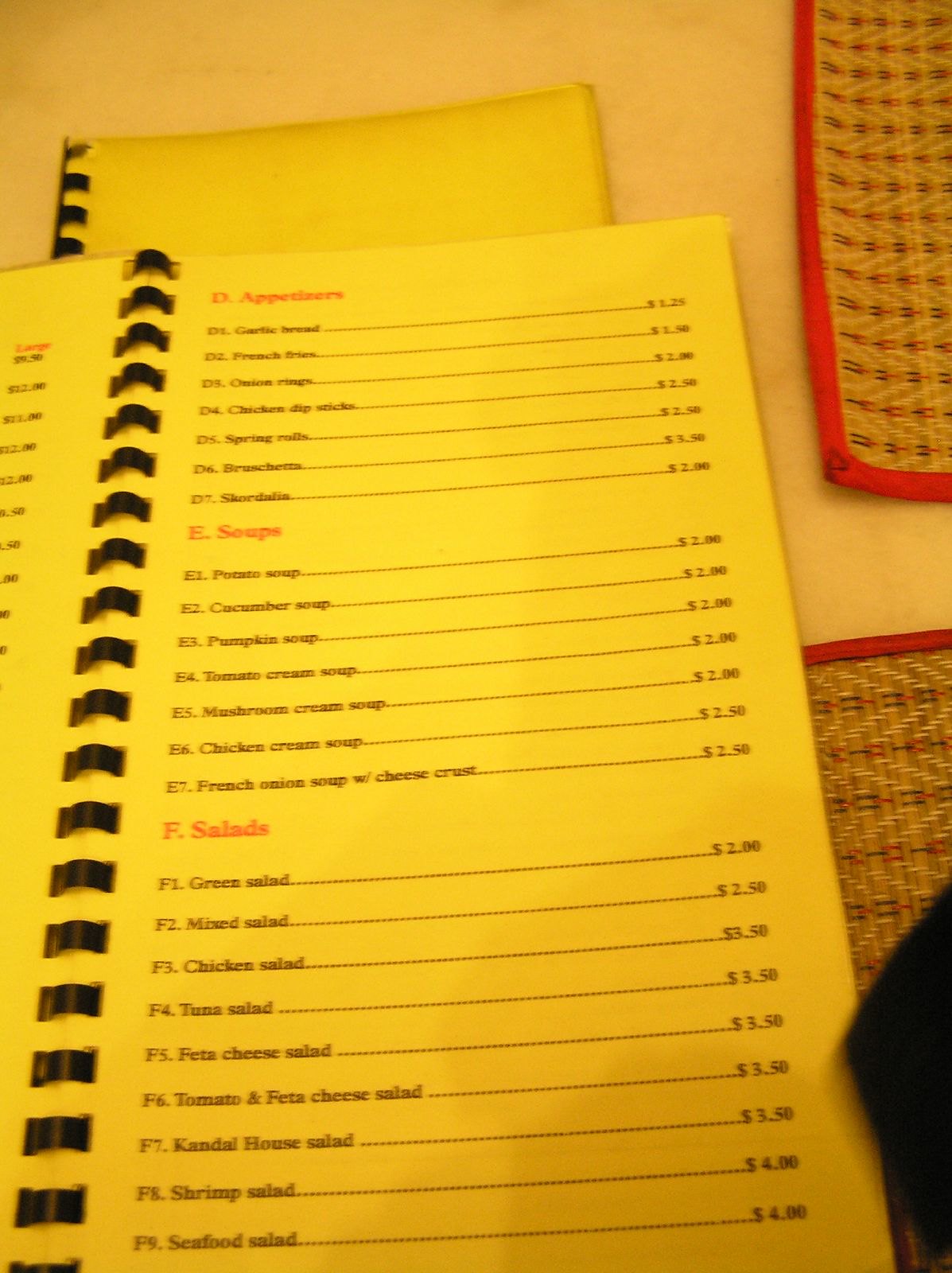This slightly out-of-focus, vertical color photograph features a notebook or a long cookbook with black spiral binding down its center, laying open with the left page cut off by the edge of the image. Beneath this, a folded menu with identical black spiral binding is visible. This menu is closed but shows three sections labeled "D," "E," and "F," in red type, which appear to correspond to appetizers, soups, and salads, respectively. Item names with a line running across separate them from their prices listed in the right column of the page. 

Flanking the cookbook/menu setup are two pieces of cloth that resemble pot holders, embellished with beige and red tones and bordered in red. Additionally, a black, indistinct object intrudes from the bottom right corner of the image. The overall hue of the photograph is a very bright yellow, indicating it was taken under artificial tungsten lighting, which casts a warm glow on the orange-yellow table surface in the background.